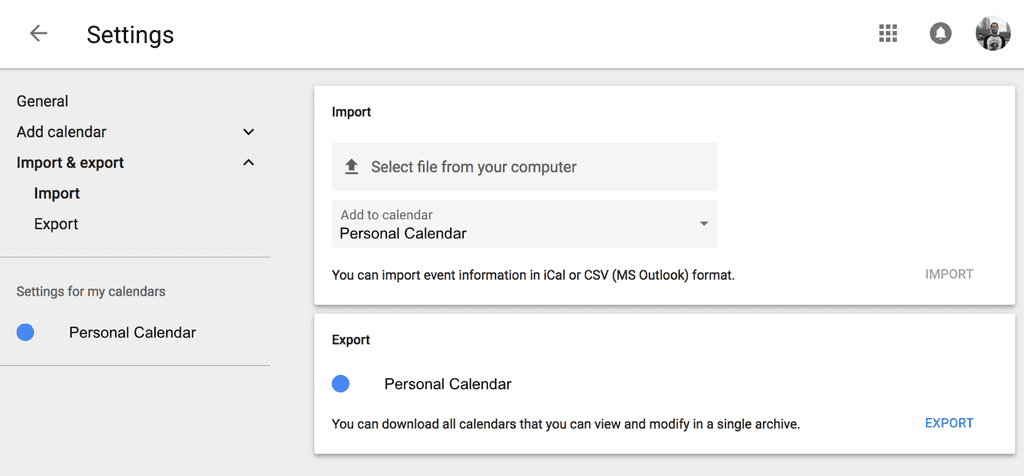The image depicts an application settings menu. At the top, a white navigation bar displays a gray back arrow to the left, the word "Settings" with a capital "S" in the center, and three icons aligned to the right: a grid of nine small squares arranged in three rows and columns, a black circle with a white bell icon, and a circular avatar of a single male posing.

Below the top bar, the interface extends into a gray background where various setting options are presented. The left section lists the settings categories. The top option is "General," followed by "Add calendar," which has a downward-pointing arrow next to it, and then "Import and export" with an upward-pointing arrow. Below these, a light gray line divides this section from "Settings for my calendars," accompanied by a blue circular icon. Under this header, there’s an option labeled "Personal calendar."

To the right side of the interface, there are two white boxes with clearly defined sections:

1. **Import Section:**
   - The top-left corner of this larger white box contains the word "Import" in black text with a capital "I."
   - Below "Import," there's a gray, underlined box with an upward-facing arrow, displaying the instruction "Select file from your computer."
   - Following this input field, two additional boxes are positioned: one gray box labeled "Add to calendar" in gray text and "Personal calendar" in black text, with a downward-pointing arrow next to it.
   - A line of black text at the bottom explains, "You can import event information in ICAL or CSV (MS Outlook) format."
   - To the right, there is an "Import" button in capital letters, which is currently grayed out and inactive.

2. **Export Section:**
   - The top-left corner of this section features the word "Export" with a capital "E" in black text.
   - Directly below "Export," a blue dot precedes the text "Personal calendar" with the initials capitalized.
   - The section includes an explanatory text informing users that they can "download all calendars that you can view and modify into a single archive."
   - In the bottom-right corner, an active "Export" button is prominently displayed in blue capital letters.

The overall layout is user-friendly, with clear separation and detailed labeling of the import and export functionalities to assist users in managing their calendar settings efficiently.